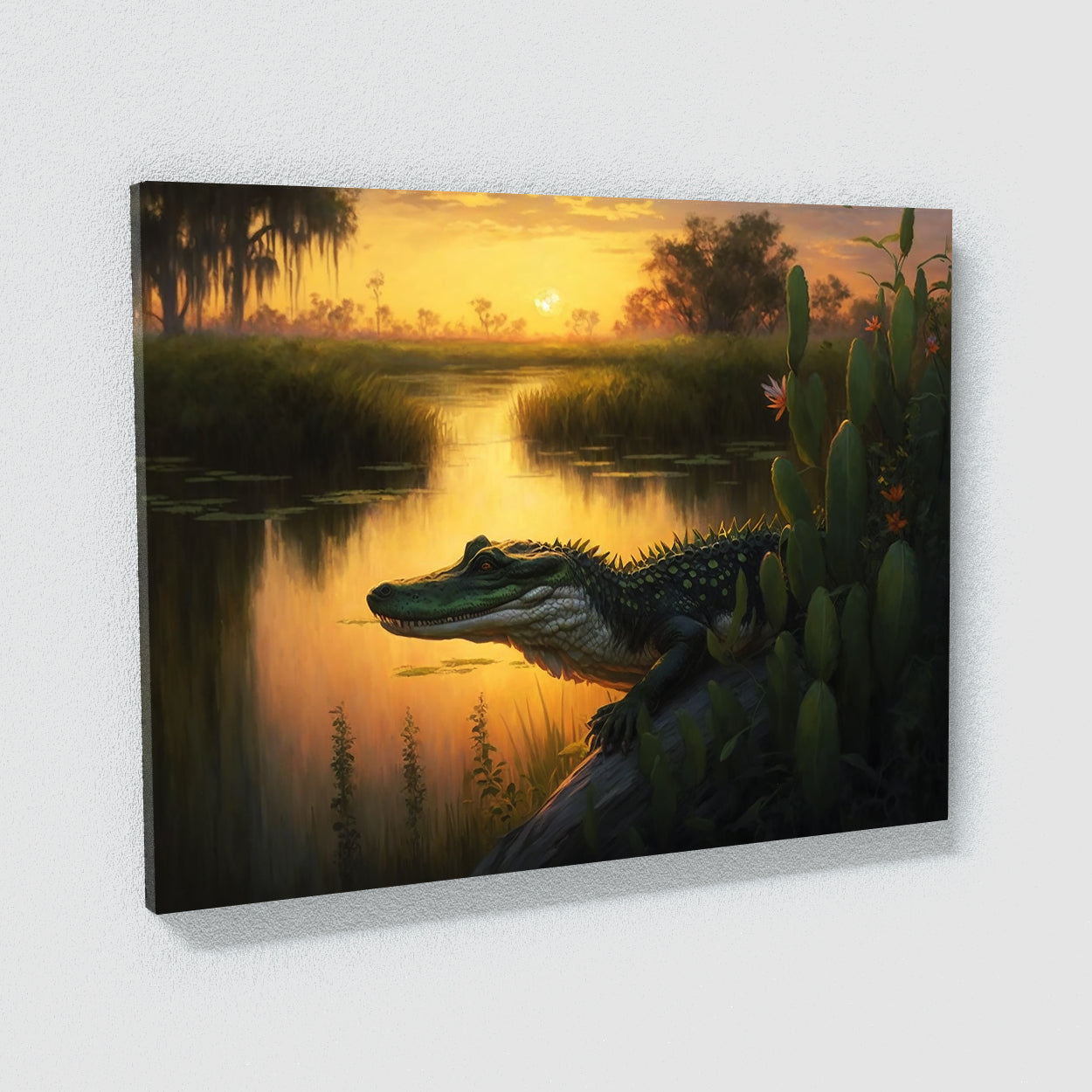This detailed painting, mounted on a gray wall, captures a serene yet wild swamp scene at sunset. Dominating the artwork is a green alligator with light green spikes and spots, white underbelly, and black eyes, perched on a rock. The alligator's rough, textured skin, scales, and claws are meticulously detailed. Surrounding the rock, the swampy landscape showcases a variety of flora, including long grass, reeds, and water lilies. A cactus stretches from the bottom right to the top right corner, adding an interesting element to the marshy environment. In the distance, tall swampy trees are silhouetted against a vibrant yellow sky, which reflects brilliantly on the water, bathing the scene in warm, golden hues. This evocative piece is offered for sale, capturing the essence of a tranquil yet untamed wetland.